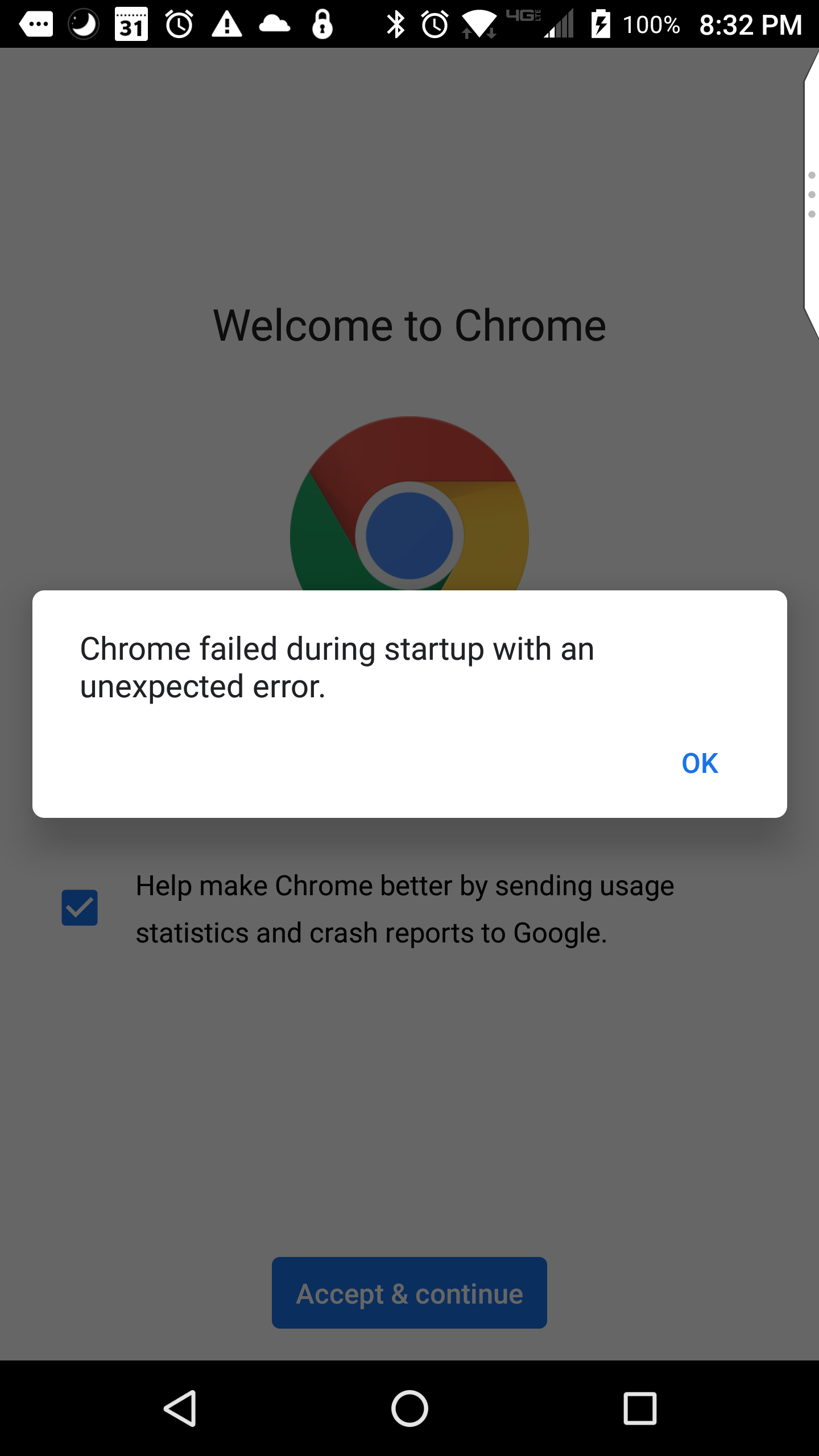This image is a detailed screenshot from a non-iPhone smartphone, displaying the upper notification bar and a Chrome browser interface. The top banner of the screen is black, filled with various icons that indicate the user's active and background activities. There are icons showing an open calendar, an alarm, a moon symbol for possibly Do Not Disturb mode, a triangle with an exclamation point signifying a warning or alert, cloud storage, a locked padlock indicating device security, Bluetooth activation, another alarm, 4G connectivity, and a battery icon showing a full 100% charge with the phone currently charging. The time shown is 8:32 PM. 

In the main part of the screen, the background image reads "Welcome to Chrome" with the Chrome logo, a multicolored circle. There is a checkmark next to a box indicating the user has opted to send usage statistics and crash reports to Google. Below this, a blue button reads "Accept and continue."

However, a pop-up message overlays this welcome screen. The pop-up is white and states, "Chrome failed during startup with an unexpected error." Below this message is an option in blue text labeled "OK," which the user can press to dismiss the pop-up.

At the very bottom of the screen, there are three navigation icons: a left-pointing arrow, a circle, and a square, typically used for navigating within the phone's interface.